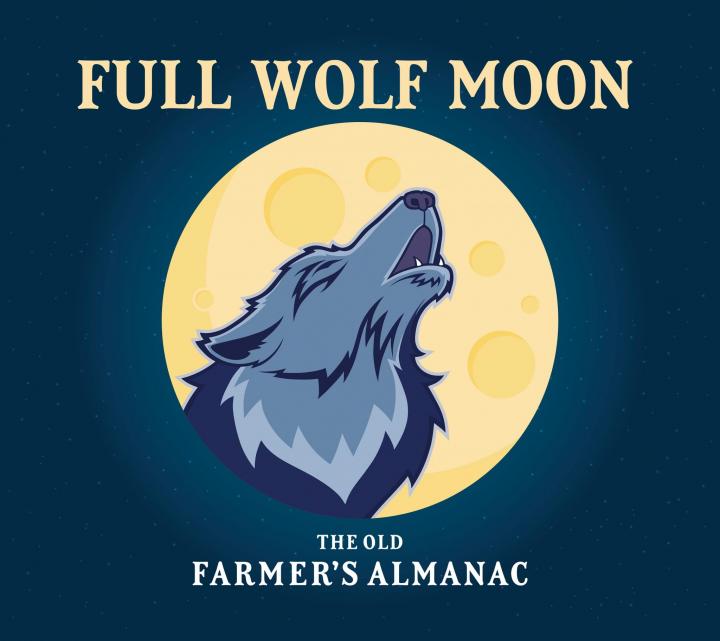The image is a squared banner intended for a blog or book, featuring a blue background speckled with small white dots that represent stars. At the top, in yellow serif text, it reads "Full Wolf Moon," and at the bottom, in white serif text, it reads "The Old Farmer's Almanac." Dominating the center, a yellow circle with multiple orange-yellow craters symbolizes the moon. Superimposed on the moon, there's a detailed cartoon rendition of a howling blue wolf, which sports a dark navy-blue mane and three shades of blue on its body. The wolf's sharp bottom teeth and open mouth add a sense of animation to the image.